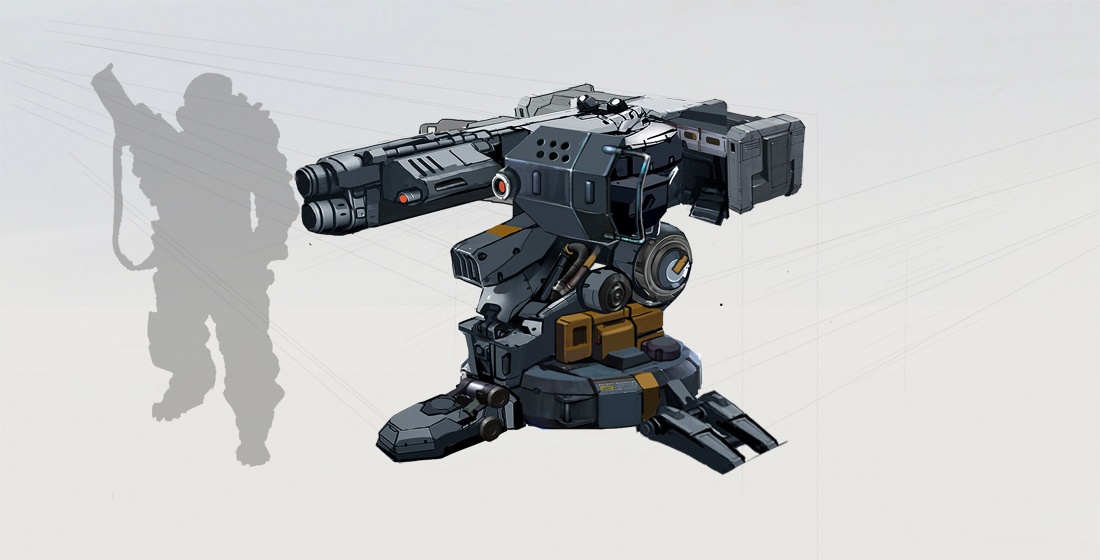The image features an intricate artist's sketch set against a light grey background, depicting a powerful, double-barrel machine gun known as the Cerberus Turret from the video game Battle for Utopia. This imposing black weapon has distinctive red dots and brownish areas, with a long strap for carrying and a base that includes a foot control area and a prominent brown square. To the left, instead of the direct shadow of the gun, there is the silhouette of a figure wearing military fatigues, equipped with a harness and holding a weapon, suggesting a soldier in a protective outfit. The detailed rendering highlights the complexity of the gun's over-and-under barrels, feeding mechanism, and aiming motors, illustrating its formidable presence as a video game turret.